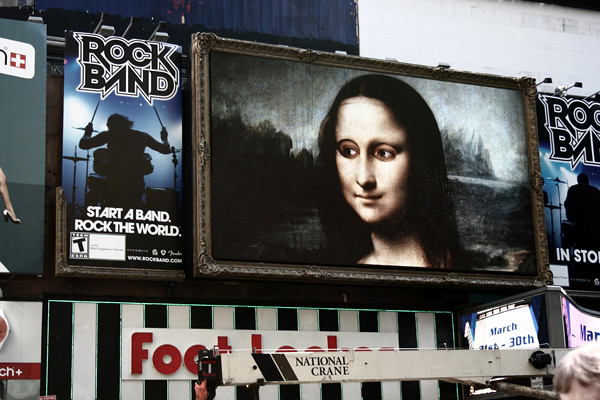The image is a detailed photograph capturing an eclectic wall inside a lively venue, possibly a restaurant with live music. Dominating the center of the wall is a horizontally framed, modernized portrait of the Mona Lisa with black hair, smiling, and facing left, set against a backdrop of black mountains, rocks, and rivers. 

Flanking this central piece are multiple rock band posters. To the left of Mona Lisa's frame, there is a tall poster with a brown frame, featuring the text "Rock Band" in black and white at the top. Below this title, a person is depicted playing drums with their arms raised, holding two drumsticks, accompanied by the words "Start a band, rock the world" in white, along with some blurry text beneath.

Below the Mona Lisa, there's a sequence of layered elements starting with black and white vertical stripes, mostly covered by the red "Foot Locker" logo set on a white background. Towards the bottom, a horizontal white and gray crane labeled "National Crane" in black letters spans the image, adding an industrial touch to the scene.

Additionally, on the right side of the image, there is another rock band poster with text, likely saying "rock band" again, and below it, a separate poster announcing an event from March 21st to 30th in blue lettering.

All these elements are mounted on the wall of what appears to be an industrial-style building, contributing to the overall bustling and creative atmosphere of the space.